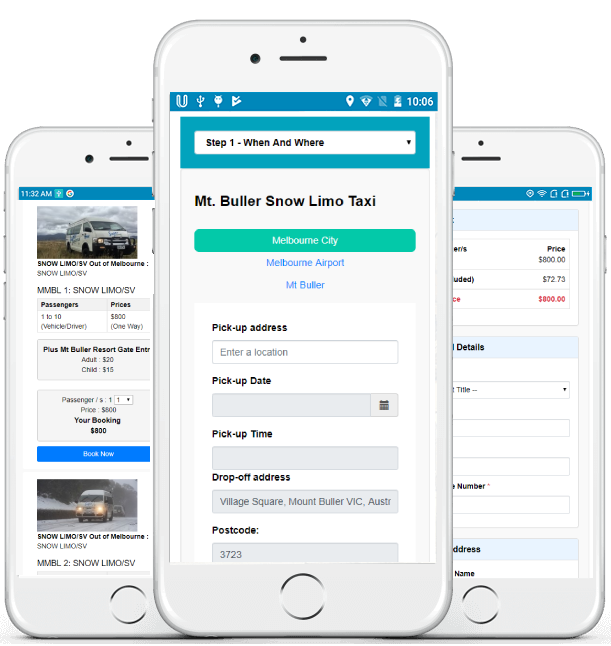The image displays three screens on a smartphone, aligned one above the other. The top screen features a drop-down menu titled "Step One: When and Where." Beneath this, the text reads "Mr. Buller Snow Limo Taxi." A teal box displays "Melbourne City," followed by a blue hyperlink labeled "Melbourne Airport." Additionally, there are input fields for "Pick Up Address" with a prompt to "Enter a location," and "Pick Up Date."

The middle screen shows an image of a van driving through a snowy street, accompanied by the word "Snow" and a descriptive caption beneath it. A blue box is also visible, although its content is not specified.

The bottom screen on the left contains a visual of a van and what seems to be a receipt. The receipt shows the word "Price" with a number beneath it, appearing to be $800. There are smaller, less visible numbers below, including one in red that is barely legible.